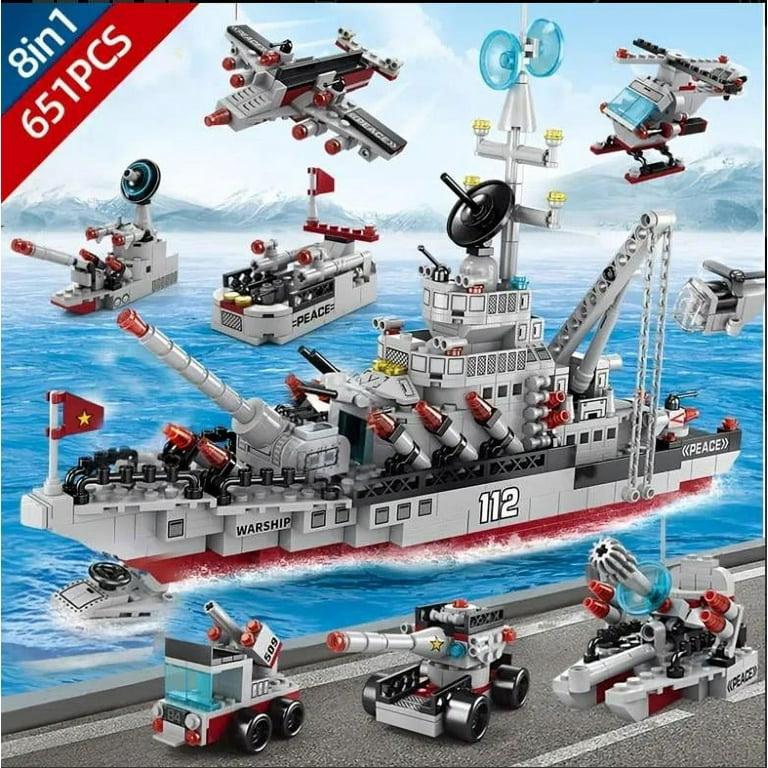This square image serves as the cover for a box of Lego-style toys, depicted as a vibrant advertisement. In the top left corner, a blue triangle with the white font reads "8-in-1," accompanied by a red stripe stating "651 PCS." The central focus combines artistic drawings and photo cutouts, showcasing various military-oriented toys. A prominently featured gray battleship is set against an ocean backdrop, complemented by smaller armed boats. Additionally, there’s a jet fighter plane, an attack helicopter, and a smaller helicopter seemingly landing on the ship. On the foreground landscape, three vehicles include a tank, a possible fire truck with a hose, and an artillery unit, each detailed with black wheels and red tips. Though not branded as Lego, the toys clearly emulate the iconic block style and are intended for assembling multiple configurations from the 651 pieces provided.